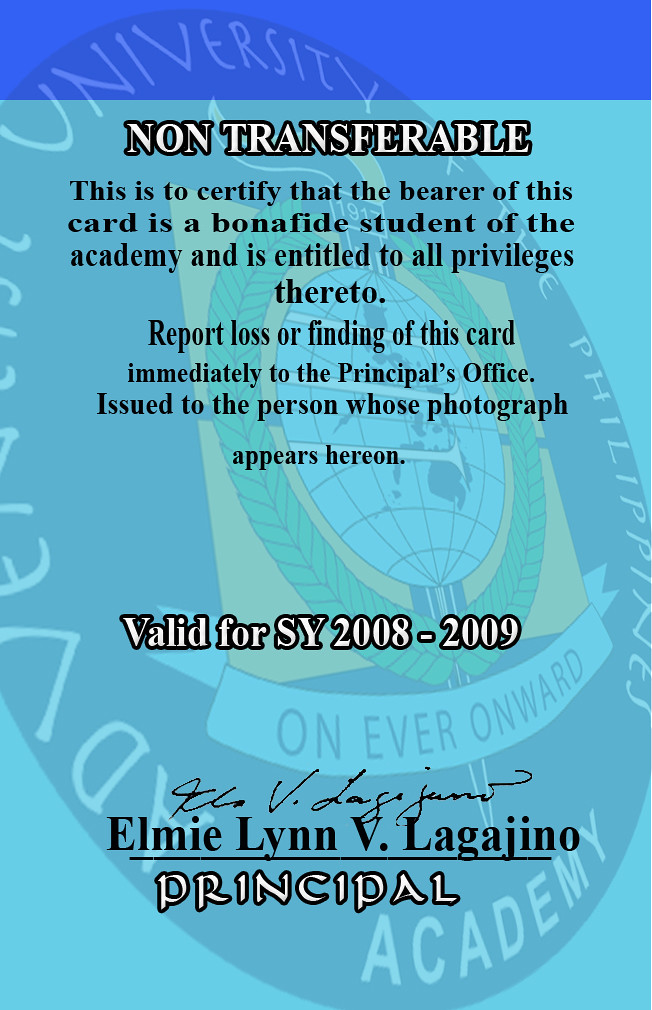The image displays a student identification card set against a blue background, featuring a detailed design. A darker blue banner spans the top with white lettering declaring the card as "non-transferable." Below, in black letters, it certifies that the bearer is a bona fide student of the Academy with access to all associated privileges. There is a stipulation to report any loss or finding of the card immediately to the principal's office. The card is issued to the individual whose photograph should appear on it, but in the image, the photograph section is blank. The validity of the card is marked as "SY 2008-2009." At the bottom, the card is signed by Elmy Lynn Lagajino, noted as the principal. A watermark featuring the Academy's emblem, a globe with the motto "Onward Ever Onward," is prominently seen in the background, tilted and semi-transparent.